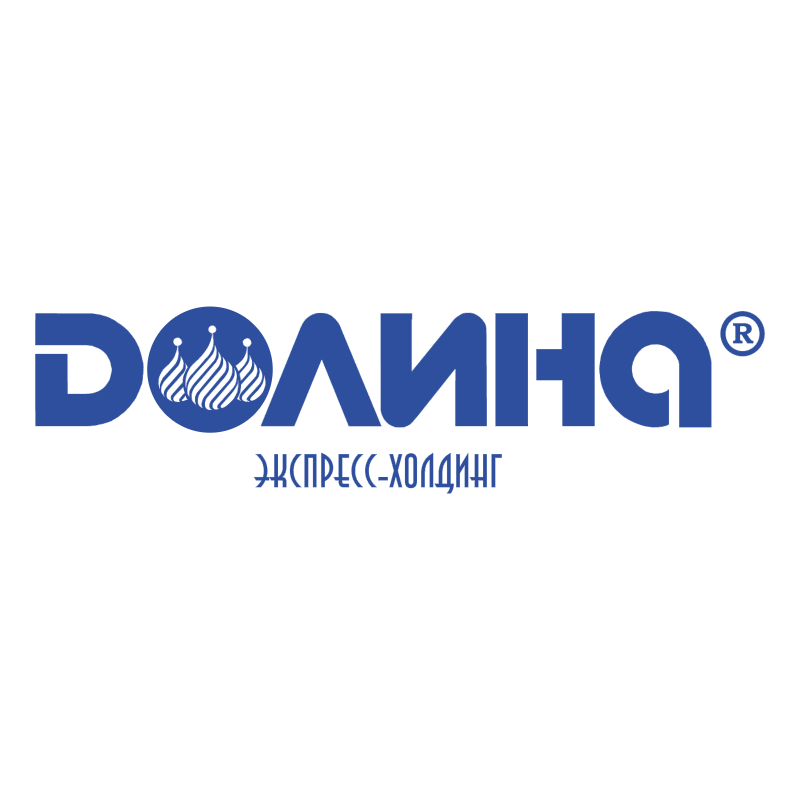The image features a centrally positioned logo on a completely white background, which provides a stark contrast to the bold blue text. The text appears to spell out "DOANA," though it is written in a language that may resemble Russian or another Cyrillic script, as there are additional subtitles in a similar script beneath the main text. The letter "O" in "DOANA" is particularly distinctive, containing three white shapes that evoke the iconic and historical onion-dome architecture of Russian buildings, or possibly resembling festive Christmas decorations. The logo concludes with a registered trademark symbol (®) placed at the end of the text, signifying its official brand status.